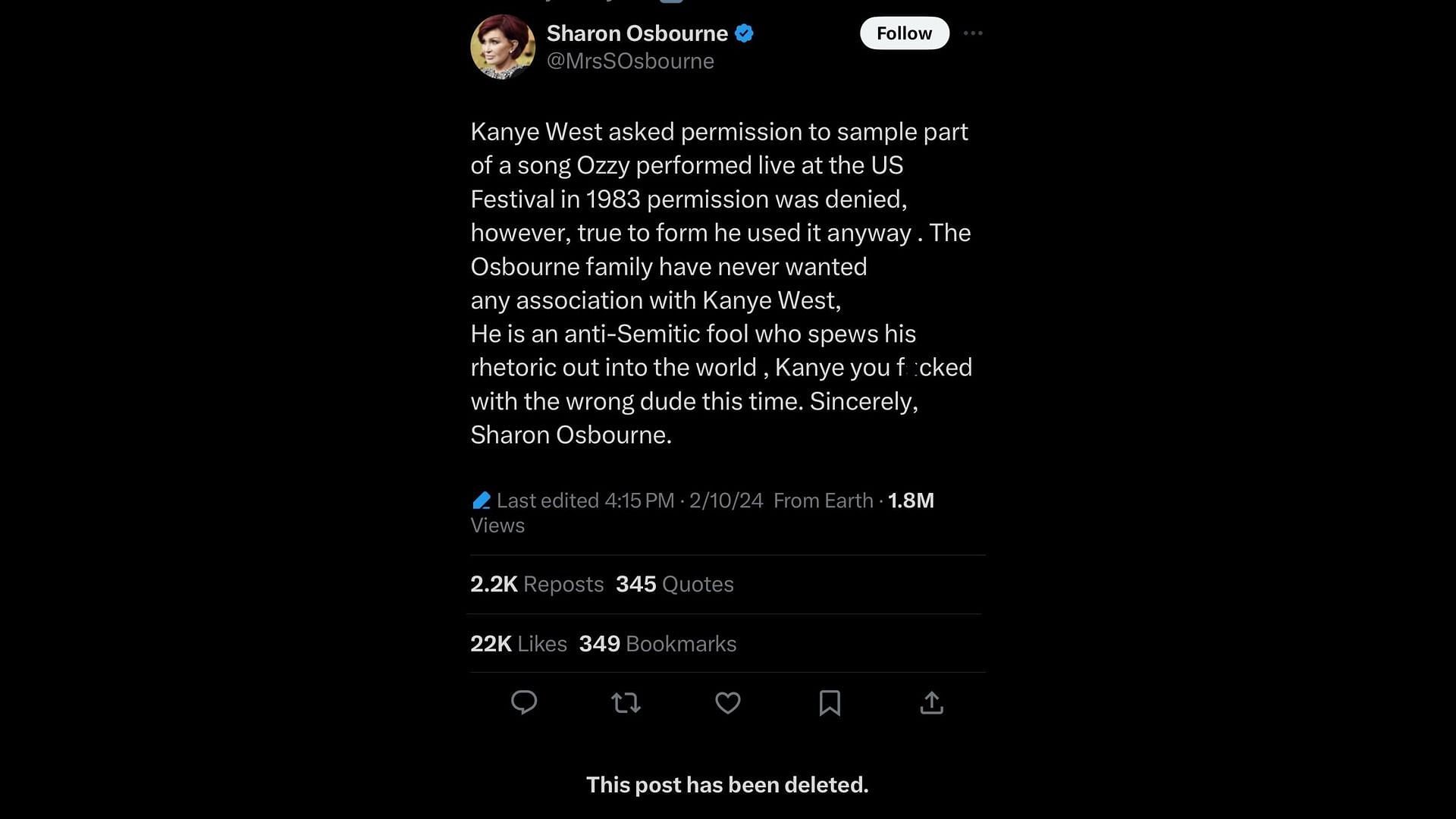The image features a prominent black background with a central circular thumbnail displaying a picture of Sharon Osbourne. Below her image, the overlay text identifies her as Sharon Osbourne, with her social media handle @MsSOsbourne, and includes a blue verification checkmark next to her name. Adjacent to her profile information, there is a "Follow" button and an icon with three dots indicating additional options.

The main body of the post relays a striking message from Sharon Osbourne regarding an incident with Kanye West. The text narrates that Kanye West asked for permission to sample a segment of a song performed live by Ozzy Osbourne at the US Festival in 1983. Despite permission being denied, Kanye proceeded to use the sample. Sharon Osbourne expresses strong disapproval, emphasizing that the Osbourne family has always distanced themselves from Kanye West, whom she labels as an "anti-Semitic fool" spreading detrimental rhetoric. The post concludes with a stern warning from Sharon Osbourne: "Kanye, you effed with the wrong dude this time. Sincerely, Sharon Osbourne."

Additional text highlights the post's metrics and status: a small blue note indicates it was last edited at 4:15 PM on October 10, 2024. The post has garnered substantial engagement with 1.8 million views, 2.2 thousand reposts, 345 quotes, 22,000 likes, and 349 bookmarks. Notably, there’s an annotation indicating that the post has been deleted. Social media interaction icons for quoting, reposting, bookmarking, and other forms of engagement are also visible.